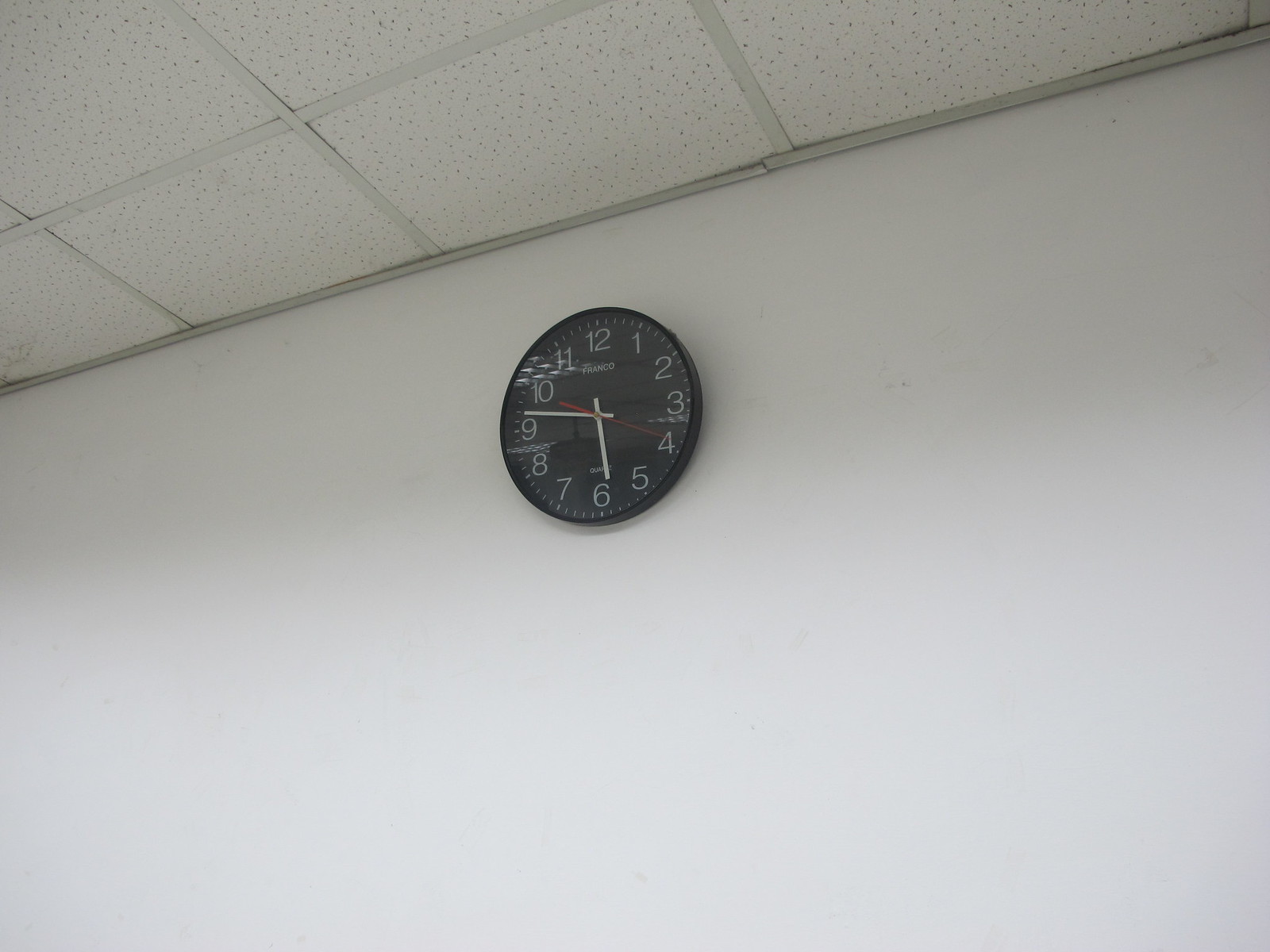In this rectangular photograph, we observe a stark white wall adorned with a round, black wall clock. The clock features a black face and rim, with prominent large white numbers. It displays the time as 5:47, with a small red second hand pointing to the 10. Above the clock, a typical drop ceiling is visible, comprised of white aluminum strips and ceiling squares. The ceiling shows signs of age, with slight unevenness and darkened edges possibly from accumulated dirt. The overall scene suggests an older building, adding a touch of character to the otherwise plain setting.